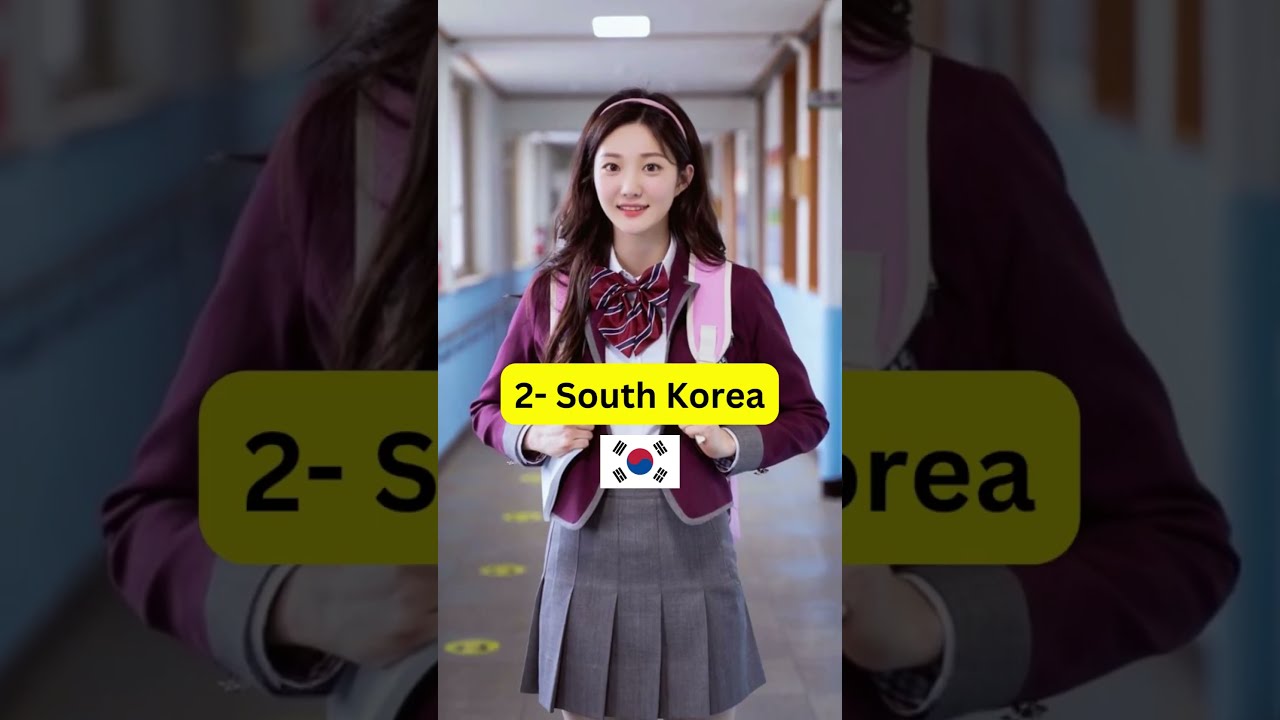In this image, we see a young Asian woman in her 20s, captured in what appears to be a still from a video. She is standing in the hallway of a school, which features a gray floor, blue and white walls, and various doors stretching down the hallway. She wears a purple or dark pink school uniform jacket over a white shirt adorned with a red and blue striped bow tie. Her outfit is completed with a gray pleated skirt. She has a pink headband holding back her dark brown or black hair and is carrying a pink backpack, identifiable by the straps visible over her shoulders. She has a confident smile on her face, and she seems to be in the middle of speaking.

Over her stomach, a yellow rectangular sign with black text reads "2-South Korea," and just below this, a South Korean flag is visible. The left and right sides of the rectangular image feature close-up, black-shaded portions of the same background sign, zoomed in to show parts of the text "2-South Korea."